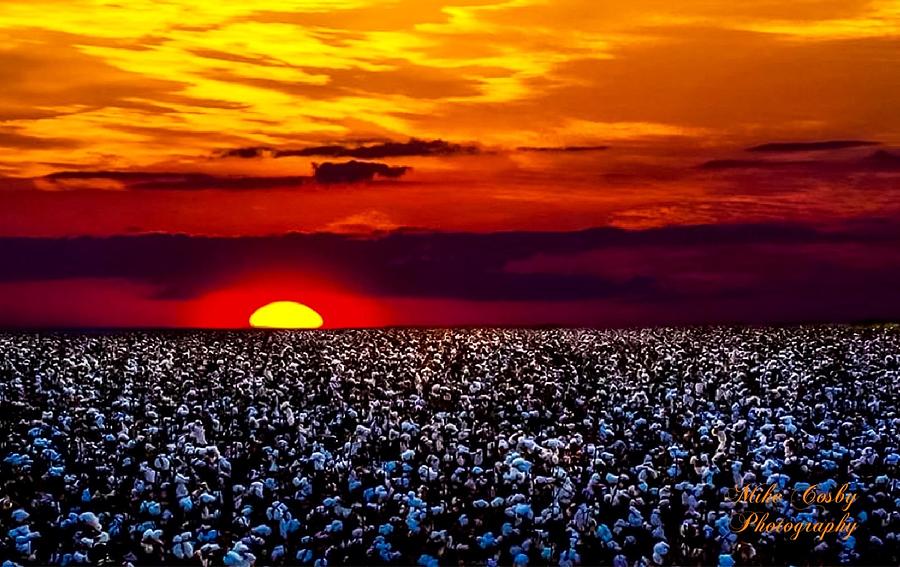The image depicts a vibrant outdoor sunset with a strikingly fiery night sky. The brilliant orange and reddish hues dominate the horizon, with the sun positioned slightly left of center, radiating a bright orange and yellow glow. Dark and bright orange clouds add depth, some of them casting stark, black silhouettes as they approach the illuminating sunset. The sky transitions from a lighter yellow at the top to a deeper red closer to the horizon.

Below the dramatic sky, a vast field extends across the bottom 40% of the image. This field is covered with blue and purple foliage, possibly flowers or plants, standing out against darker, silhouetted stalks. The field and sky are divided by a straight horizon line, creating a stark contrast between the vivid upper sky and the serene field below.

In the lower right corner, the text "Mike Cosby Photography" is elegantly displayed in cursive gold text, underscoring the artistic quality of the photograph.